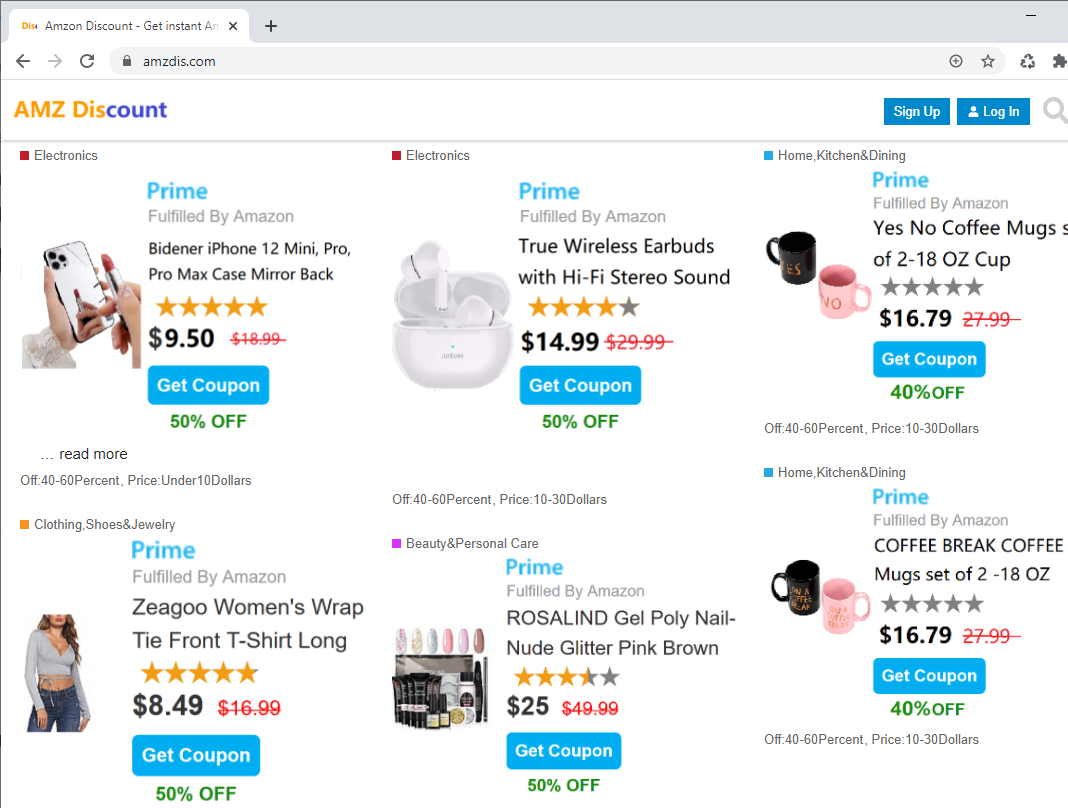This image features a webpage from a shopping website called AMZDiscount, designed to work in conjunction with Amazon. The layout comprises two rows of three items each, which together convey a somewhat low-quality aesthetic typical of budget-focused online marketplaces. Each product is marked with the label "Fulfilled by Amazon," suggesting that while the items are listed on a third-party site, their fulfillment is handled by Amazon, adding a layer of legitimacy. 

In the top left corner of the first row, there's a basic iPhone case priced at $9.50. To its right, a pair of true wireless earbuds with hi-fi stereo sound is advertised for $14.99. Completing this row are two 18-ounce coffee mugs, surprisingly the most expensive item so far, priced at $16.79.

The second row kicks off with a Zigu woman's wrap tie front t-shirt, modeled by a woman showcasing her midriff. This trendy piece of fashion is followed by a Rosalind gel poly nail set available in nude, glitter, pink, and brown shades for $25.00. The row is rounded out with a duplicate listing of the same set of coffee mugs seen in the row above.

Overall, the assortment of goods reflects a spread of inexpensive products with a mix of tech accessories, fashion items, beauty products, and everyday household items.